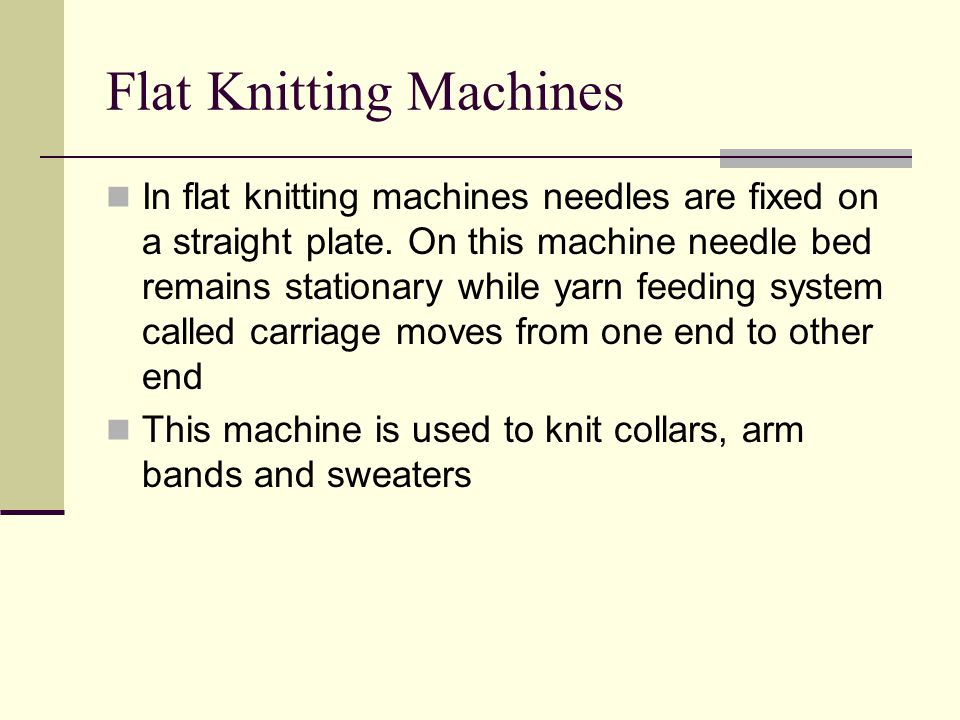The image features a PowerPoint slide with a beige or pale yellow background. On the left side, there is a dark green vertical border extending more than two-thirds down from the top. At the upper left corner, there is a black thin line running along the top, ending in a gray rectangular shape. The slide title, "Flat Knitting Machines," is prominently displayed in large black text. Below the title is an underscore line that also stretches partway through a gray rectangle covering the border. The slide contains two detailed bullet points explaining the functionality of flat knitting machines. The first point states: "In flat knitting machines, needles are fixed on a straight plate. On this machine, the needle bed remains stationary while the yarn feeding system, called a carriage, moves from one end to the other end." The second bullet point explains: "This machine is used to knit collars, armbands, and sweaters." Additionally, at the very bottom of the left border, there is a small purple edge.